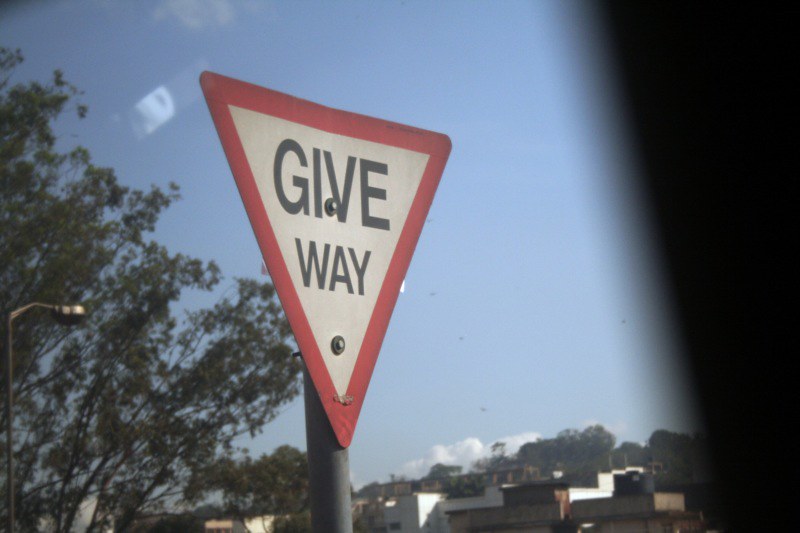The image captures a 'Give Way' sign, distinctively shaped as an upside-down triangle with a red border and bold black letters on a white background. The photo is taken from inside a car, evidenced by the visible part of the black interior on the right side. The car is moving past a mix of urban scenery that includes tree-lined streets, a streetlamp, and buildings whose rooftops and top stories peek above the horizon. The sky is a serene blue, scattered with distant clouds. The precise nature of the buildings—whether residential or commercial—remains unclear.